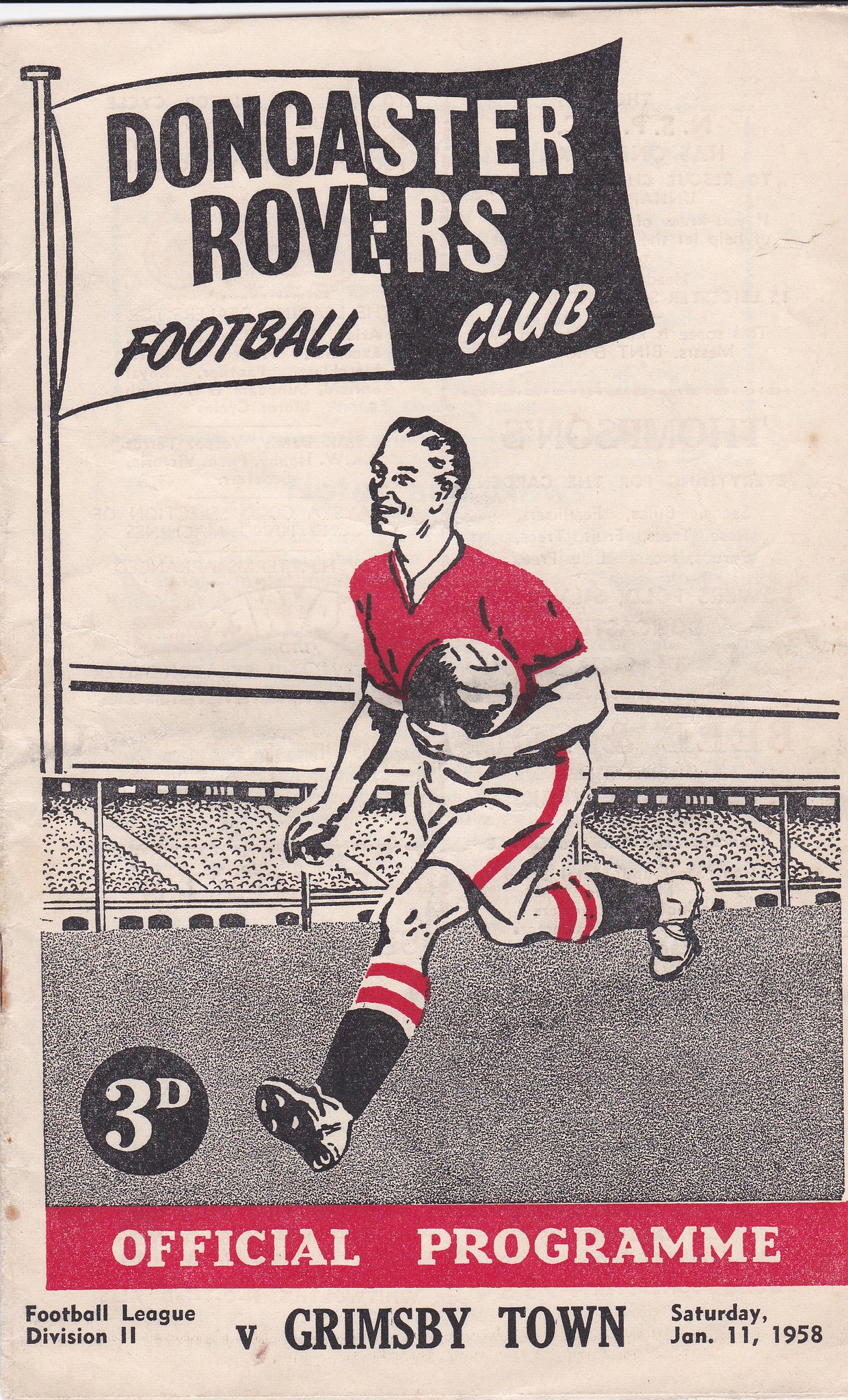The image is the front cover of an official program for a football match between Doncaster Rovers Football Club and Grimsby Town, dated Saturday, January 11th, 1958. The cover prominently features a football player in the center, wearing a red shirt and white pants with a red stripe, running with the ball across the field. Behind him, a stadium and a cheering crowd are visible. The top left corner of the cover shows the Doncaster Rovers Football Club flag. The design of the cover includes a variety of colors such as white, tan, black, red, and different shades of gray. The text on the cover states: "Doncaster Rovers Football Club Official Program Football League Division 2 vs. Grimsby Town Saturday January 11th, 1958."